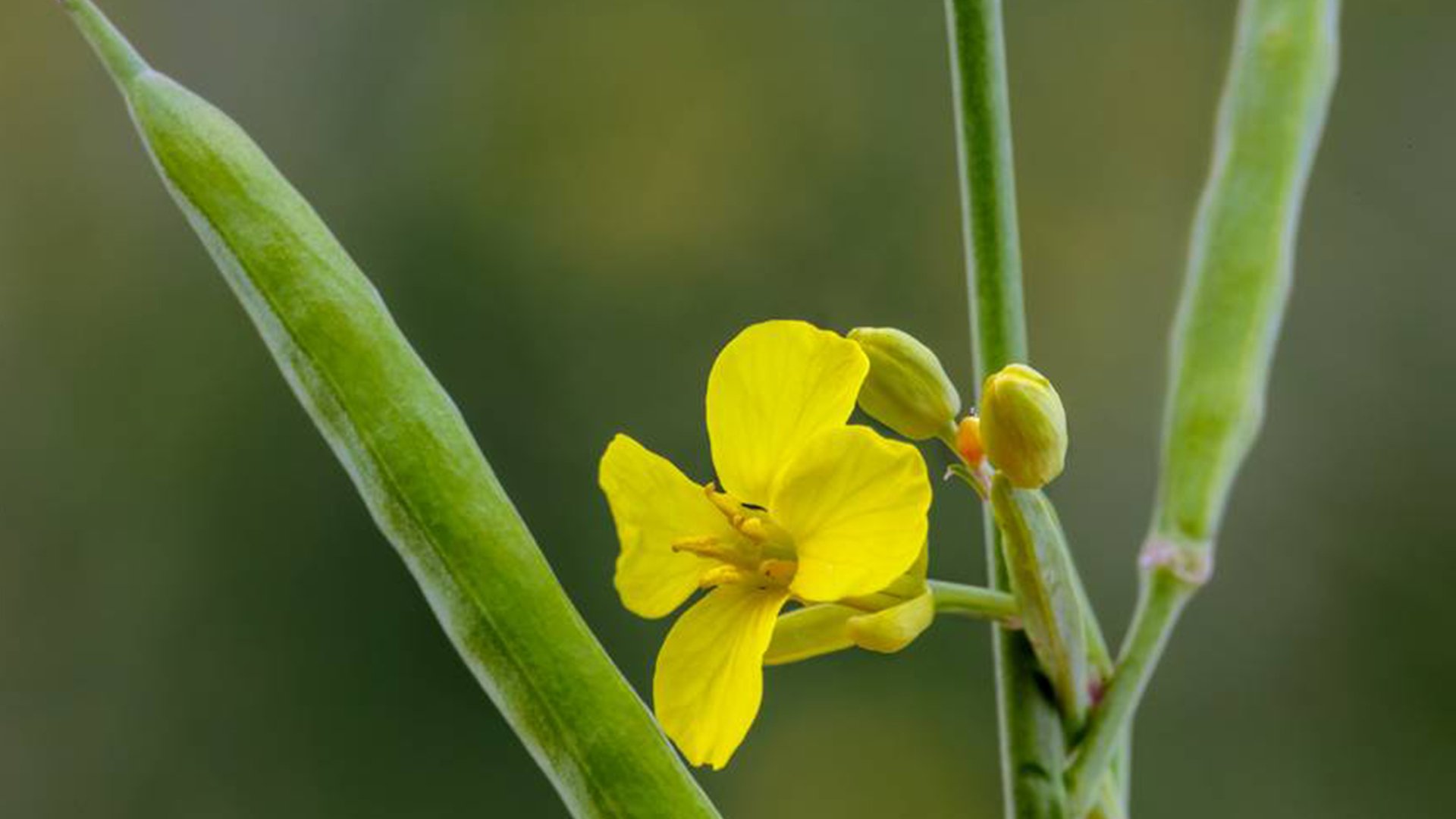This image captures an intimate close-up of a delicate yellow flower, slightly out of focus, drawing attention to its subtle details. The flower is oriented slightly to the left, revealing its intricate structure with pronounced yellow petals. At the center, the flower showcases slender, cone-shaped protrusions designed to hold pollen. It stands gracefully atop a green stalk, from which several unopened buds emerge. These buds vary in size and color, with the larger ones being predominantly green with yellow tinges, and a smaller one showing hints of orange. Surrounding the flower, multiple stems and stalks create a complex network: a prominent vertical stalk extends off to the right, a thick green stalk rises at the base of the image, and another thicker stalk resembling a bean pod ascends and exits the frame to the right. The backdrop is a nondescript, blurred mix of dark green and yellow hues, hinting at a lush environment that remains beautifully indistinct.